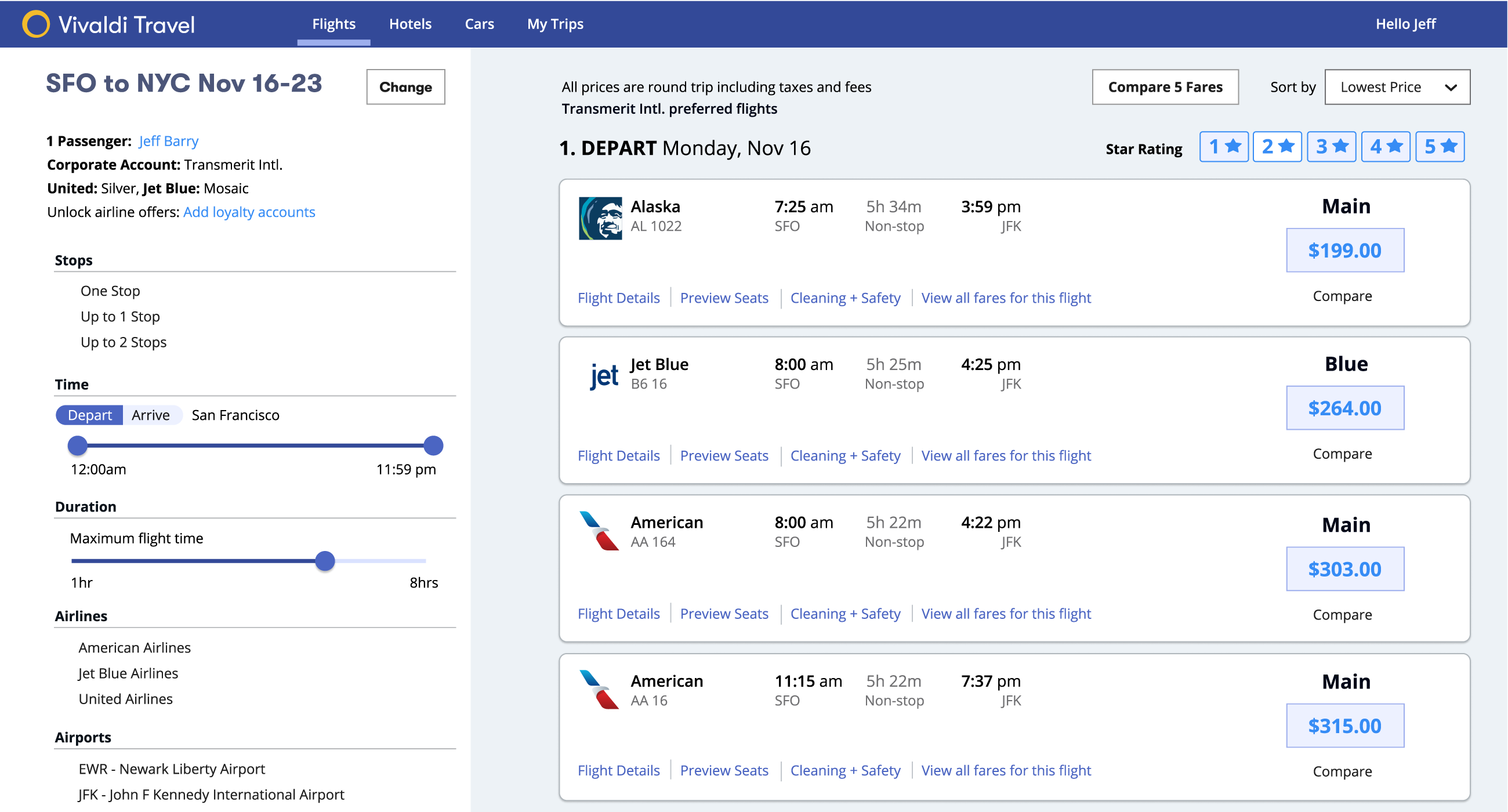The screenshot depicts a travel booking website interface, Vivaldi Travel, designed for hassle-free flight reservations. The website features a blue navigation bar at the top, with the company's name "Vivaldi Travel" presented in white font, accompanied by an orange circle with a blue center. This navigation bar includes various sections like "Flights," "Hotels," "Cars," and "My Trips," with the "Flights" section highlighted.

In the upper right-hand corner, a greeting message reads "Hello, Jeff." The interface is split into two main sections. The left section, occupying about 30% of the screen, displays a flight search box. It shows a trip from San Francisco (SFO) to New York City (NYC) scheduled from November 16 to 23 for one passenger, Jeff Barry, using a corporate account with Transmira International. The preferred airlines listed are United and JetBlue, with a filter option allowing up to two stops. Additional flight parameters include departure and arrival times, ranging from 12 a.m. to 11 p.m., and a maximum flight duration filter between 1 to 8 hours. 
      
Below, there's also a selection for preferred airlines, including American Airlines, JetBlue, and United Airlines, and airport preferences between Newark Liberty (EWR) and John F. Kennedy International (JFK).

The right section, making up about 70% of the screen, has a light bluish background and is dedicated to displaying and comparing flight options. Two main boxes are visible—one to compare fares and another to sort by criteria, with the current selection set to "Lowest Price."

A detailed flight list is presented under "Depart Monday, November 16th" with a star rating system and four chosen flights. These flights include:
- Alaska Airlines: Departs at 7:25 AM, arrives at 3:59 PM at JFK, priced at $199.
- JetBlue: Departs at 8:00 AM from SFO, arrives at 4:25 PM at JFK, priced at $264.
- Two American Airlines options: 
  - First: Departs at 8:00 AM, arrives at 4:22 PM, priced at $303.
  - Second: Departs at 11:15 AM, arrives at 7:37 PM, priced at $315.

Each flight box contains pricing details, flight duration, and departure/arrival information, allowing users to compare and select their preferred option easily.